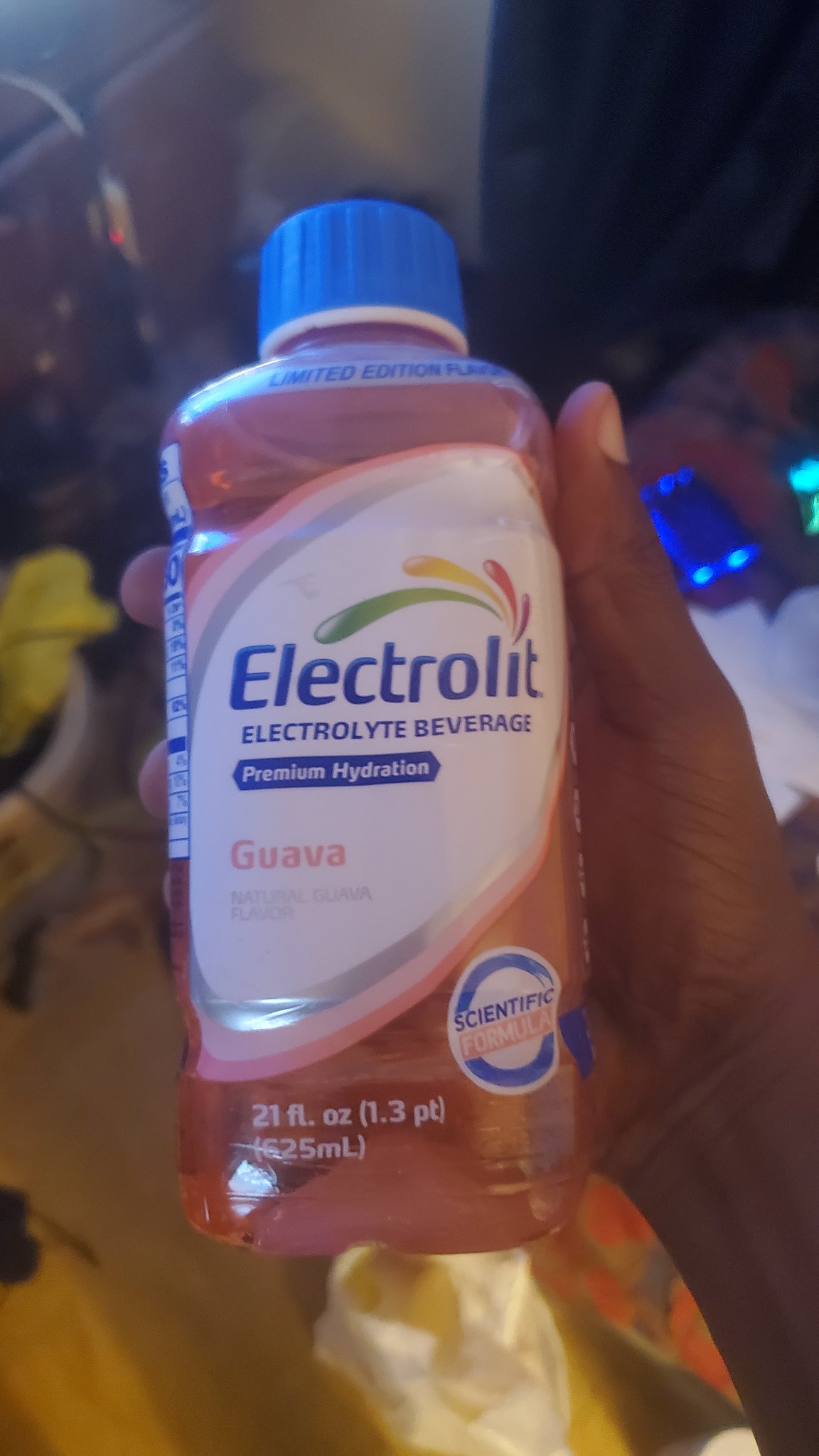This image showcases a right hand with dark skin holding up a clear plastic bottle of a beverage. The bottle features a light blue plastic lid and a detailed label. The prominent blue letters on the label spell "Electro-Lit, Electrolyte Beverage," accompanied by a design of colored teardrops emanating from the word "Electro-Lit." Below this, a blue banner with the words "Premium Hydration" stands out. Additionally, the label has "Guava" written in striking pink letters, indicating the flavor of the light pink liquid inside. Further down the label, a circular emblem with a white background and blue border reads "Scientific Formula," adding an element of credibility and assurance to the product.